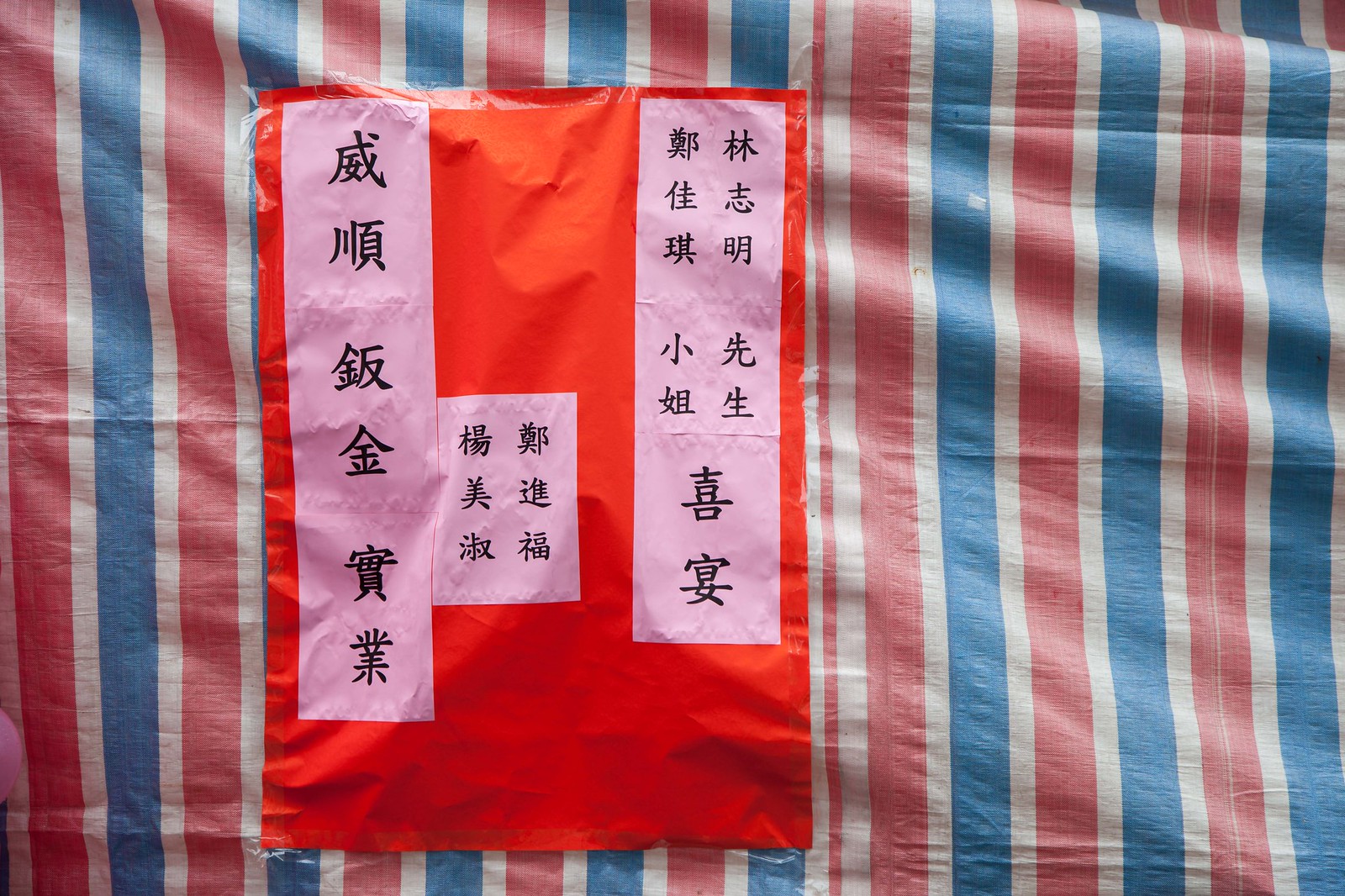The image features a wavy, cloth-like background comprising vertical stripes in a repeating pattern of wide red, narrow white, and blue stripes with some lighting and shadowing effects. Taped or affixed to this colorful backdrop is a large, red, rectangular poster or tarp made from what appears to be thin plastic or construction paper. The poster is noticeably wrinkled, suggesting it could be flapping in the wind. On the poster, there is a series of bold, black letters that appear to be either Chinese, Korean, or Japanese, likely Japanese kanji, arranged vertically. The text is divided into three distinct panels: a longer one on the left, a shorter panel in the middle, and another lengthy panel on the right, slightly shorter than the one on the left. The central part of the poster and the surrounding striped fabric are illuminated in such a way that you can almost detect a light source behind them, creating a striking and vibrant visual effect reminiscent of a carnival or circus advertisement.